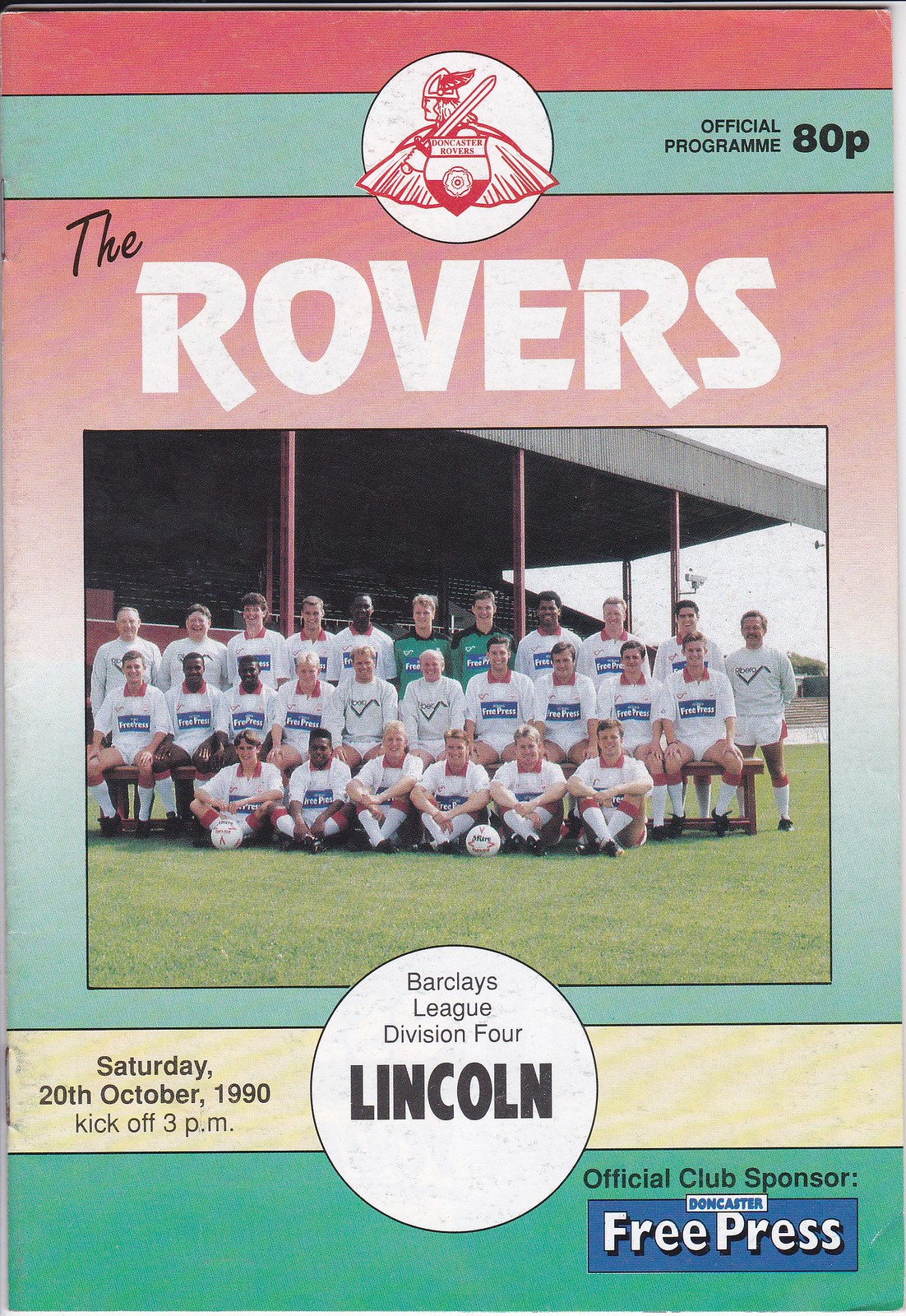The image depicts a vintage cover of a program for a soccer match, featuring Doncaster Rovers. The cover displays a colorful gradient background, transitioning from red at the top, through white in the middle, to green at the bottom. At the very top, there is a prominent logo in a white circle, illustrating a Viking warrior holding a sword behind a red and white shield labeled "Doncaster Rovers." To the right of the logo, the text "Official Program ATP" is printed within the green strip. Below this, in bold, stylized white letters, the headline reads "The Rovers."

The main subject is a team photograph set against a soccer field, with visible audience stands and the stadium in the background, bathed in daylight. The team is arranged in three rows: six players sit on the ground with two footballs in front, ten players are seated on a middle bench, and eleven players stand behind. All are dressed in white jerseys except for two individuals in the top middle row who are wearing green jerseys.

At the bottom of the photograph, a yellow horizontal strip includes the details of the match, stating "Saturday, 20th October 1990, kickoff at 3pm." Centrally positioned within this strip, another white circle denotes "Barclays League, Division 4, Lincoln," with “Lincoln” emphasized in large, bold black font. Finally, on a green strip at the bottom right corner, "Official Club Sponsor Doncaster Free Press" is highlighted, with "Free Press" encased within a blue rectangle and "Doncaster" in a smaller white rectangle just underneath. The overall design and details reflect the era and significance of the event.